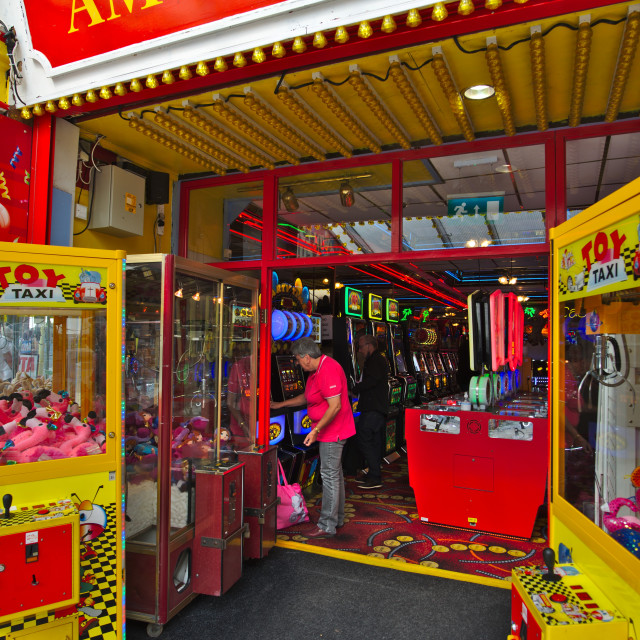The image showcases a vibrant, retro-style arcade with both outdoor and indoor elements. At the storefront, a red sign with the partially visible text "AM" is displayed against a backdrop of strip lighting, creating a nostalgic 1970s to 1990s ambiance. Flanking the entryway are two yellow claw machines labeled "Toy Taxi," featuring glass fronts with various items inside. Inside the arcade, a colorful psychedelic carpet sets the scene, reflecting the multitude of colors in the space including red, yellow, orange, black, gray, green, and blue. A woman, possibly an attendant or a player, is seen at the front, wearing an orangey-pink shirt, blue jeans, and a pink bag, engrossed in one of the arcade games. The interior is bustling with scattered gaming machines and a general air of lively chaos, consistent with the arcades typically found in beachfront or tourist locales.